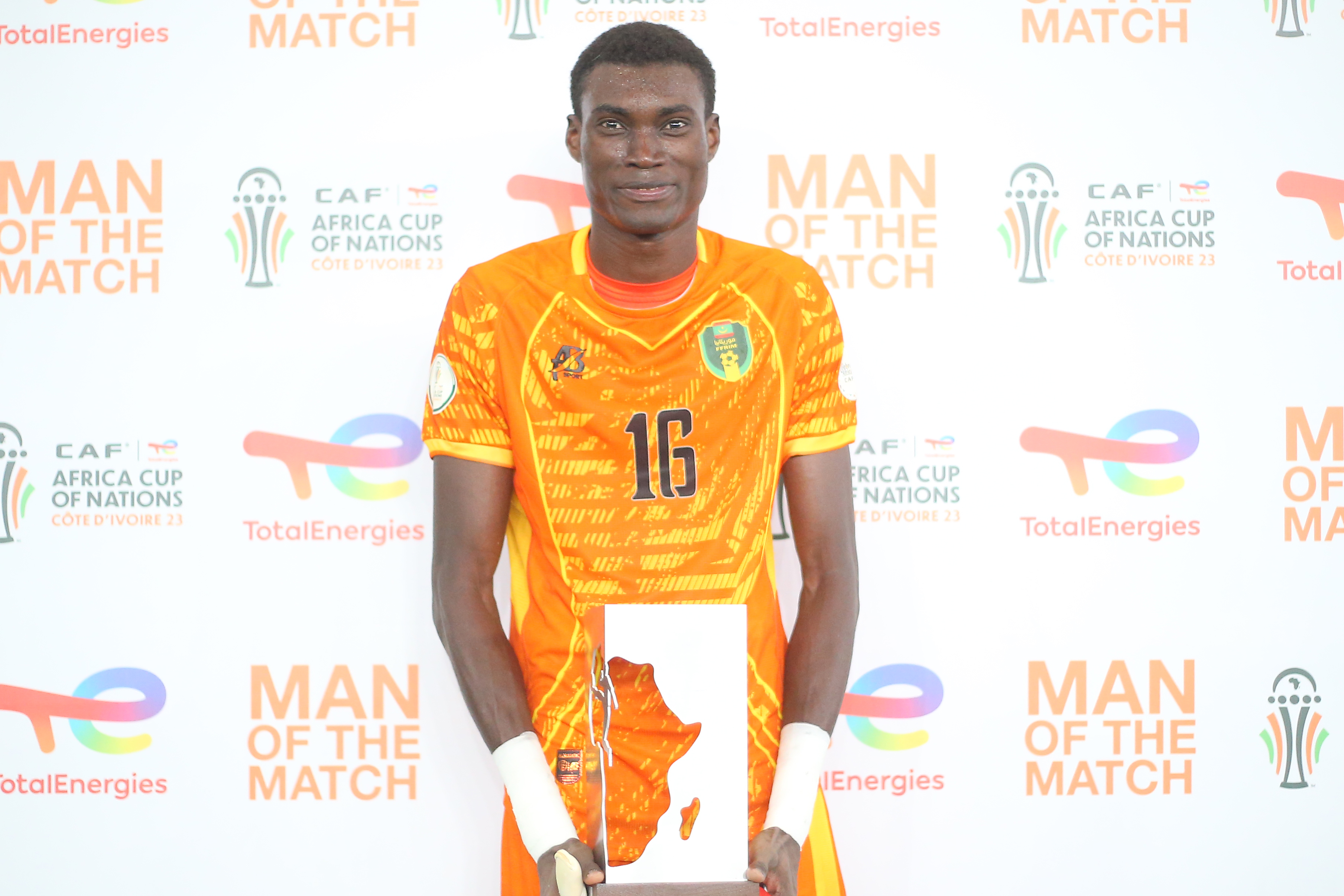This photograph captures a young Black man, standing proudly in front of a Total Energies-sponsored white backdrop decorated with logos and text for the CAF Africa Cup of Nations. The athlete, who has short hair and is clean-shaven, is donning an orange soccer uniform adorned with yellow stripes and the number 16 on his chest. His right side sports a captain's patch bordered in green and light green. The athlete's uniform, including his short soccer pants, features intricate patterns of orange and gold. High up on his forearms are white wristbands, with one of his fingers also wrapped, possibly due to an injury. Positioned centrally in the photo area labeled "Man of the Match," he holds a distinctive white rectangular trophy with a cutout shape of Africa, symbolizing his remarkable performance in the tournament. The backdrop further emphasizes the significance of the event with repeating logos and the title "Man of the Match" prominently displayed.